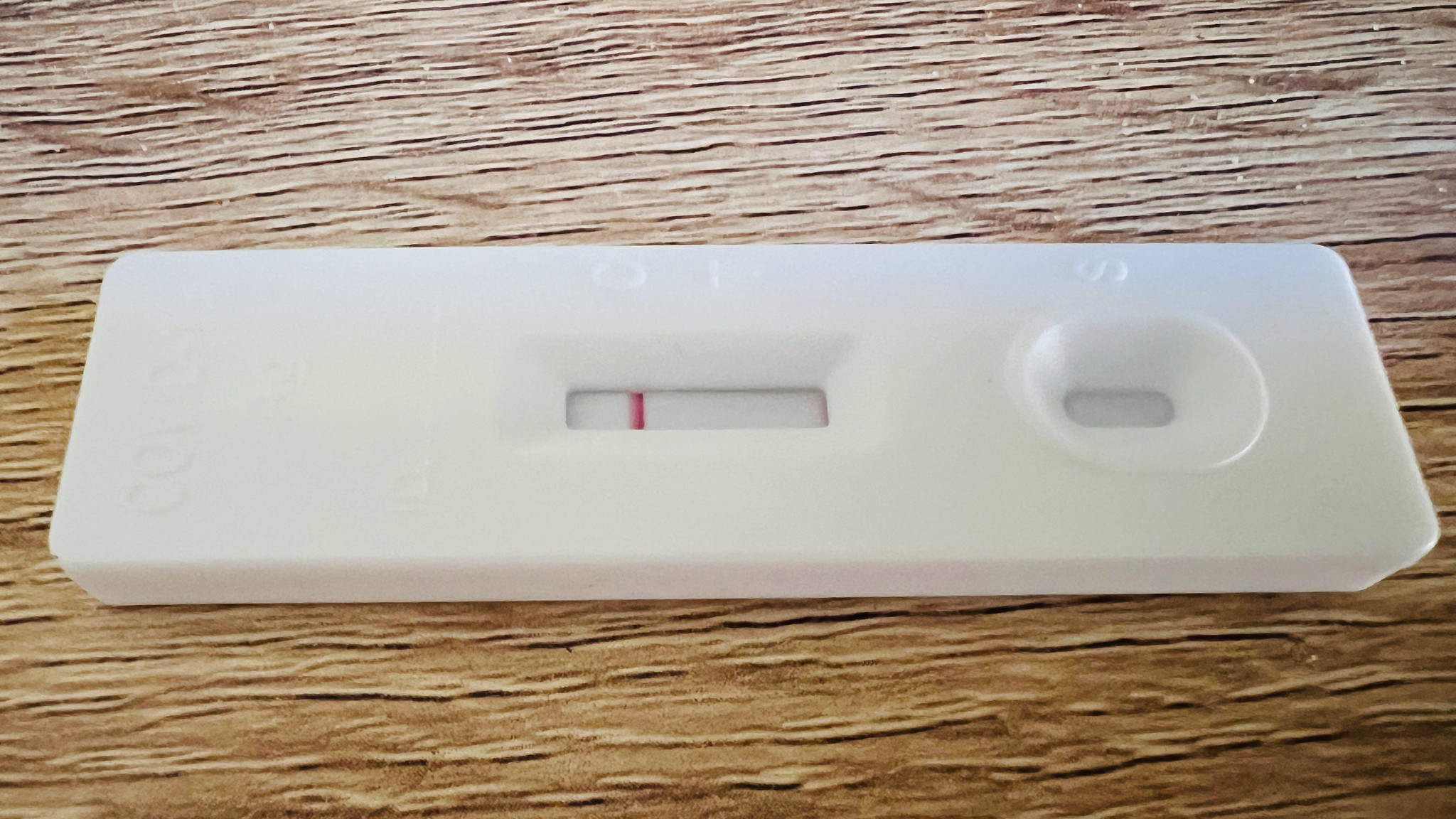The image showcases a detailed close-up of a COVID-19 rapid test. The test itself is a substantial, white, rectangular plastic stick, prominently positioned on a faux wood table surface, clearly exhibiting a laminate wood grain pattern. Notably, white specks are scattered across the top right and top left corners of the table, adding texture to the setting.

The test reveals one red vertical bar in the readout area, indicating a negative result for COVID-19. On the left side of the test, there is a long, rectangular window; this is the section where the results are displayed, signifying whether the test is positive or negative. 

Adjacent to this, on the right side, is a small oval-shaped indentation encircled by a pressing oval border. This area is the designated spot for applying the solution. The raised edges around this indentation ensure that the solution is properly absorbed into the test. The overall composition of the image is meticulous, highlighting both the functional aspects of the test and the textured context of its placement.